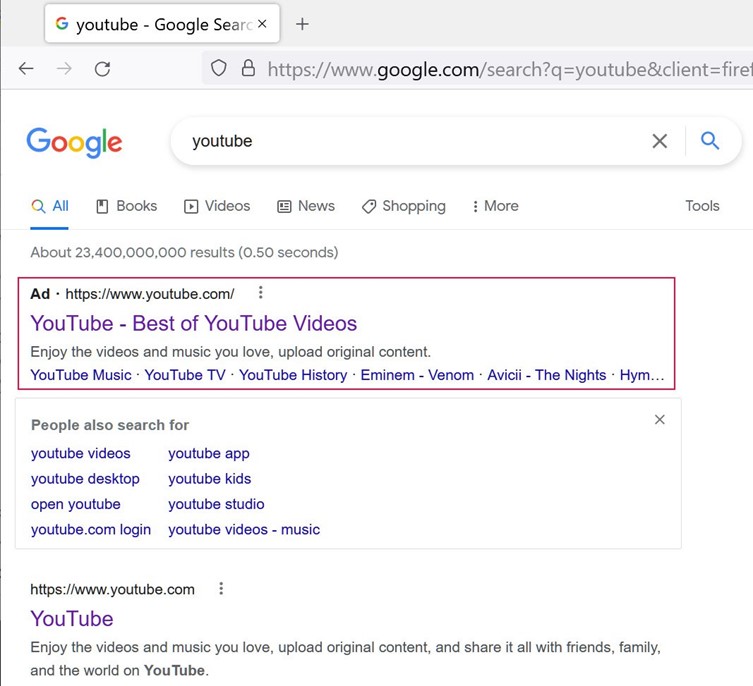A screenshot captures a Google search results page. The iconic Google logo is prominently displayed in the top left and top right corners of the browser window. The browser's single open tab showcases the Google search engine interface. The search query yields approximately 23,400,000,000 results in just 0.5 seconds. Highlighted within these results is a text snippet that reads, "YouTube, best of YouTube videos."